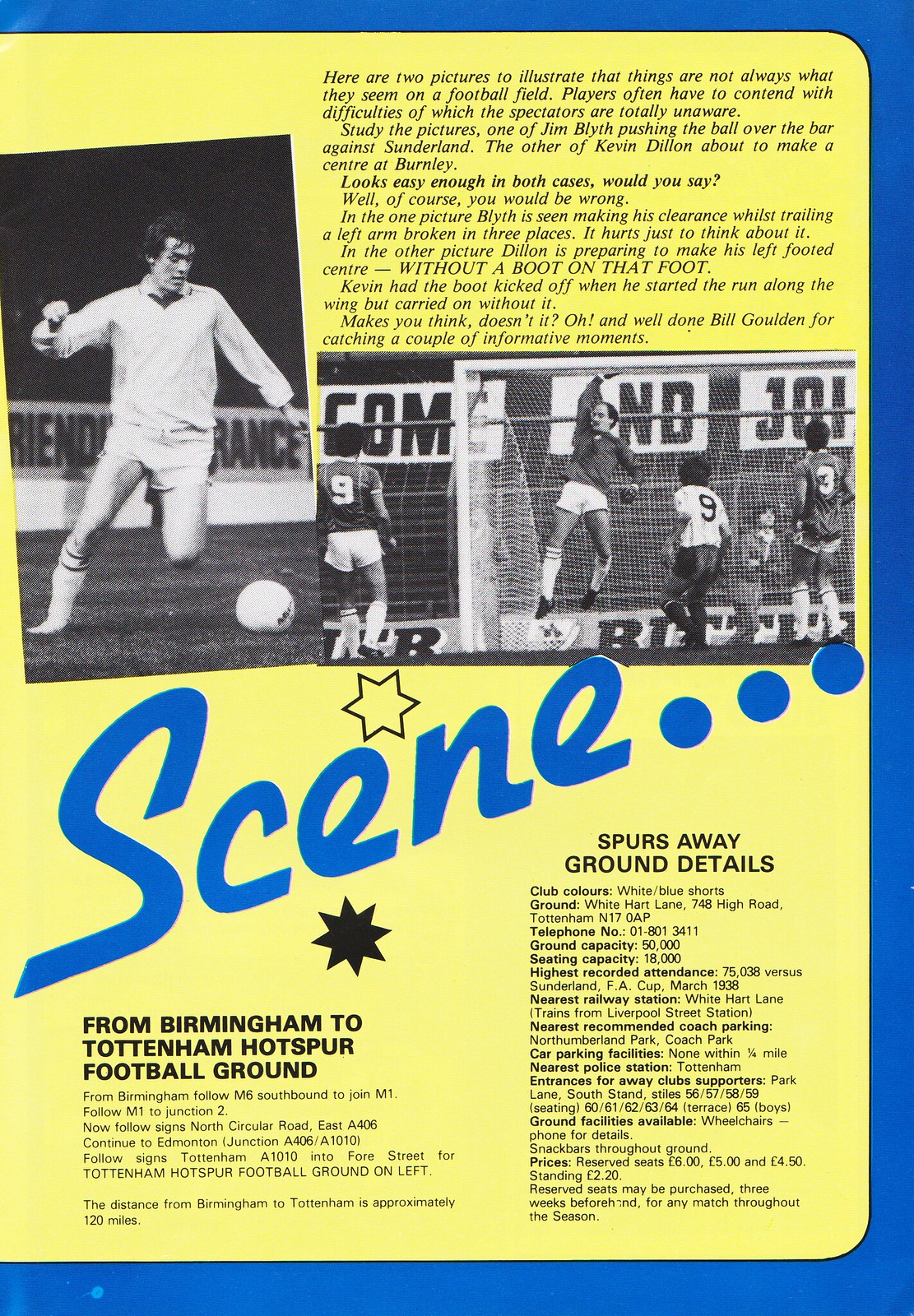The image depicts a page from an old soccer program, featuring a predominantly yellow background with blue framing along the top, bottom, and right edges, and accented by black text. The main headline reads "SEEN" in large, prominent letters, with the subheading mentioning "From Birmingham to Tottenham Hotspur Football Ground" and "Spurs Away Ground Details."

Central to the page are two black-and-white photographs capturing intense moments on the football field. The first image shows Jim Blythe pushing the ball over the bar in a match against Sunderland, despite having a left arm broken in three places. The second photograph depicts Kevin Dillon about to make a center at Burnley, astonishingly without a boot on his left foot, having had it kicked off during his run along the wing.

A small paragraph at the top of the image elaborates on these action shots, emphasizing how players often deal with challenges unseen by spectators. The bottom of the page is dense with detailed information about the away ground, including a long list of statistics covering ground capacity, seating arrangements, parking, facilities, prices, and ticket purchasing options. Specific details about the stadium include reserved seat prices ranging from four and a half to six pounds, standing tickets at 220, and the availability of reserved seats three weeks before any match throughout the season.